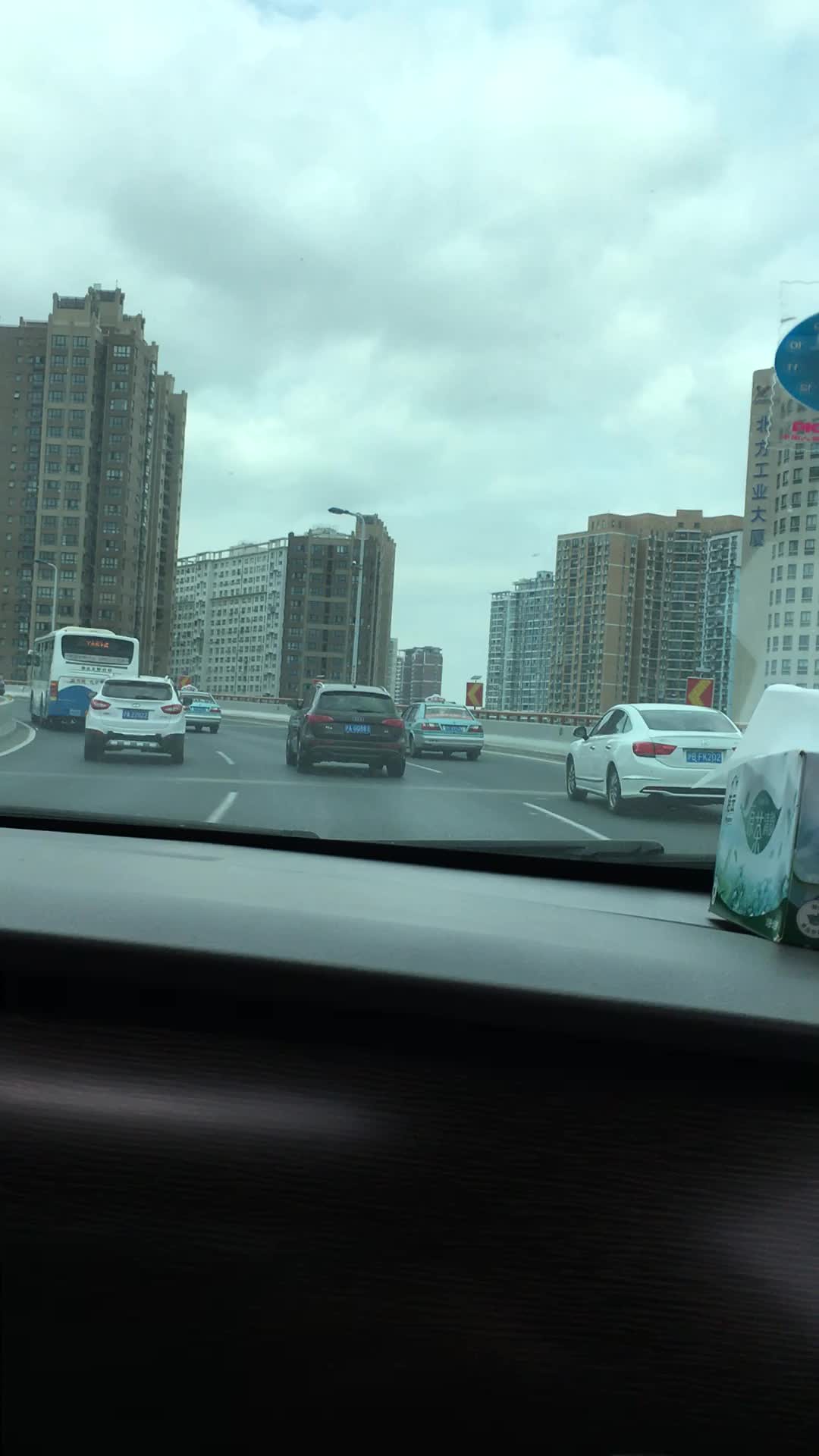The photo, a realistic vertical rectangle, captures a view from the passenger seat of a car traveling over a three-lane highway overpass. The dark dashboard of the vehicle, lighter on top, features a tissue box in the bottom right corner. The road, composed of gray asphalt with white lines, is populated by several vehicles: a black SUV, two white cars (one an SUV, the other a sedan), a silver car, and a sixth indistinguishable vehicle. Additionally, there is a white and blue bus visible on the left. The scenery outside suggests daytime with a light blue sky partly obscured by clouds suggesting imminent rain. Skyscrapers, including one with Chinese lettering, stand tall in the background, hinting that the location might be in China.